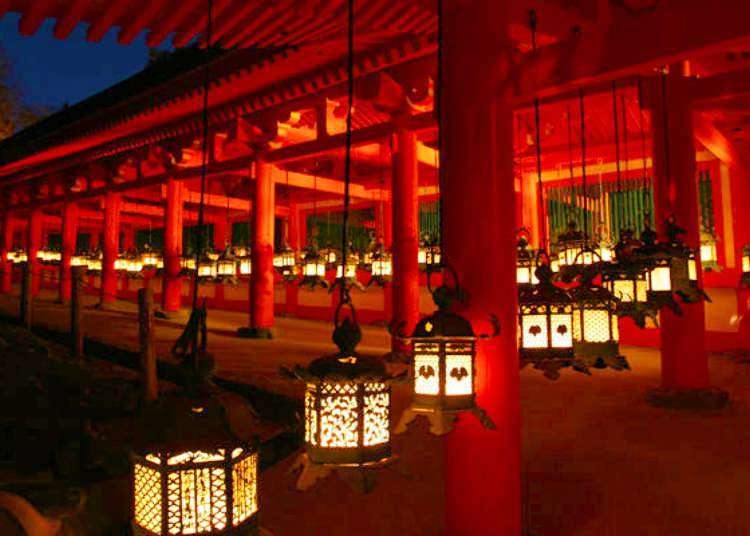The nighttime photo captures an enchanting scene of a traditional Japanese shrine, characterized by its open, airy design and intricate wooden structure. The shrine features numerous pillars supporting the roof, creating a sense of grandeur and architectural elegance. The absence of defined walls allows for an unobstructed view of the night sky in the upper left corner, emphasizing the serenity of the setting.

A prominent pathway, appearing as an L-shaped walkway, is visible in the foreground. It ascends diagonally towards the upper right corner before making a sharp 90-degree left turn, continuing into a long, inviting hallway. This pathway is flanked by a series of hanging lanterns, which outline the perimeter with their warm glow. These lanterns, made of black metal and emanating a yellow light, cast a comforting, fire-like hue that paints the wooden pillars and shrine in shades of red, orange, and yellow. This illumination creates a cozy, ember-like ambiance, enhancing the shrine’s inviting atmosphere.

Even though the surrounding greenery is barely visible due to the night, the focus remains on the lit-up structure, where the detailed arrangement of the lanterns almost touching each other complements the consistency and symmetry of the open hallways. The entire scene exudes a warm, inviting glow, making the shrine appear both tranquil and majestic in the stillness of the night.